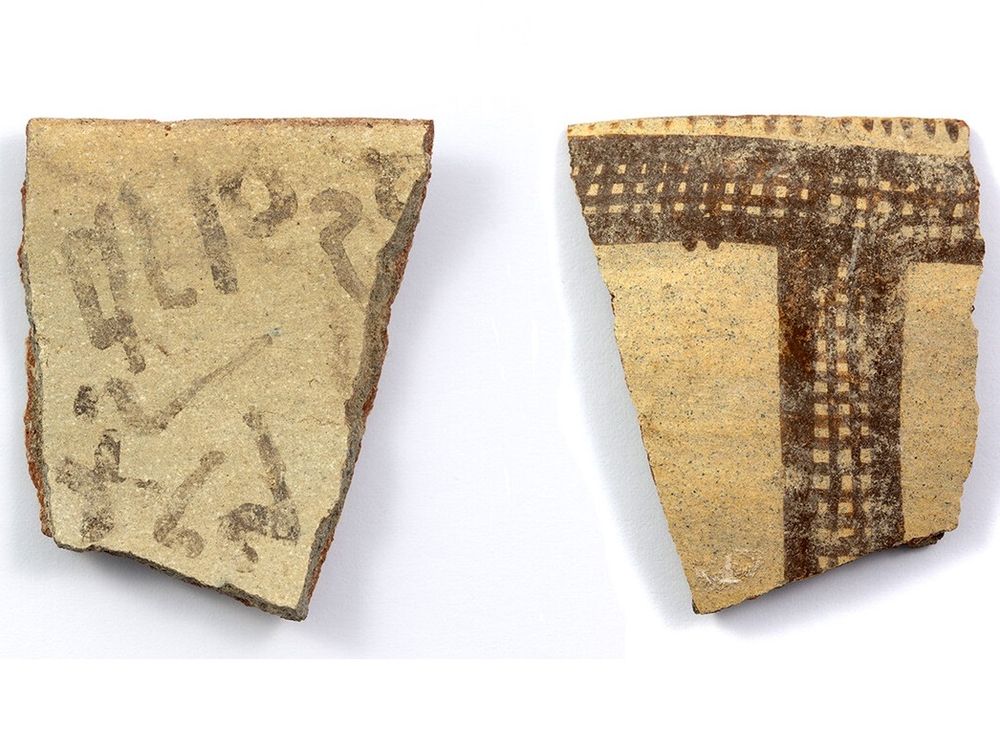The image showcases two ancient relics, possibly shards of sandstone or clay from a larger artifact like a pot or a wall, that have been unearthed through paleontological excavation. Both pieces exhibit jagged, broken edges indicative of their fragmented state and age. They feature a tan-colored base with a speckling of darker pigments, including black and reddish-brown.

The fragment on the left is adorned with various cryptic graphics that may represent an ancient alphabet or series of check marks, question marks, and other symbols such as a "4," "L," "I," and "6." The right fragment displays a T-shaped, trellis-like pattern composed of intersecting lines, running horizontally and vertically across its surface. Overall, these relics appear to be remnants from a long-lost civilization, primarily illustrated in brown hues amid their earthy stone backdrop.